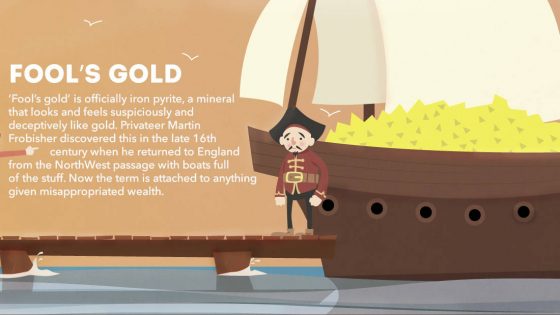The image is an informational slide featuring a detailed 2D drawing with a tan background and white squiggle lines representing seagulls. Central to the image is a very sad-looking pirate standing at the end of a dock. He is wearing a red coat and a black tricorn hat. To his right is a brown boat with white sails, filled with various yellow triangles depicting treasure. To the left of the pirate, white text on the beige background reads: "Fool's Gold. Fool's gold is officially iron pyrite, a mineral that looks and feels suspiciously and deceptively like gold. Privateer Martin Frobisher discovered this in the late 16th century when he returned to England from the Northwest Passage with boats full of the stuff. Now the term is attached to anything given misappropriated wealth." The water around the dock and boat is illustrated in shades of gray and light blue, giving a sense of location and atmosphere to the scene.